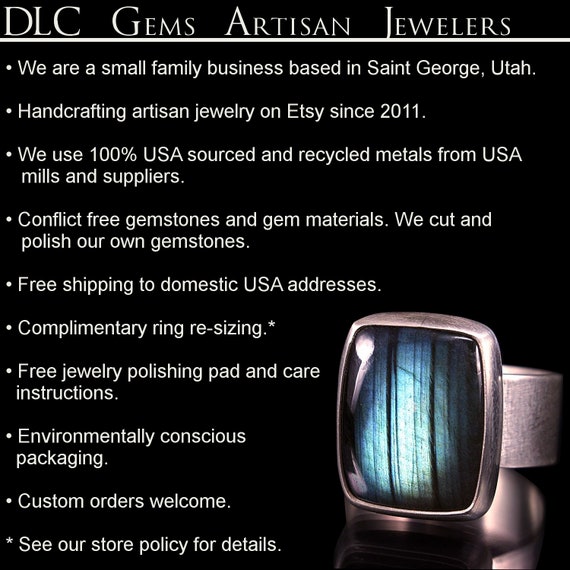The advertisement portrays a piece of jewelry against a black background, prominently featuring a ring in the lower right-hand corner. This ring is silver or pewter with a square or rectangular-shaped teal gem, streaked with black lines, creating a visually striking centerpiece. The advertisement's header reads "DLC Gems Artisan Jewelers" in white text, followed by a bulleted list detailing the company's offerings and values. They are a small family business based in St. George, Utah, and have been handcrafting artisan jewelry on Etsy since 2011. They pride themselves on using 100% USA-sourced and recycled metals from domestic mills and suppliers, use conflict-free gemstones and materials, and cut and polish their own gemstones. Additional customer perks include free shipping to domestic USA addresses, complementary ring resizing, a free jewelry polishing pad and care instructions, environmentally conscious packaging, and the availability of custom orders. The text concludes with an invitation to see their store policy for further details.